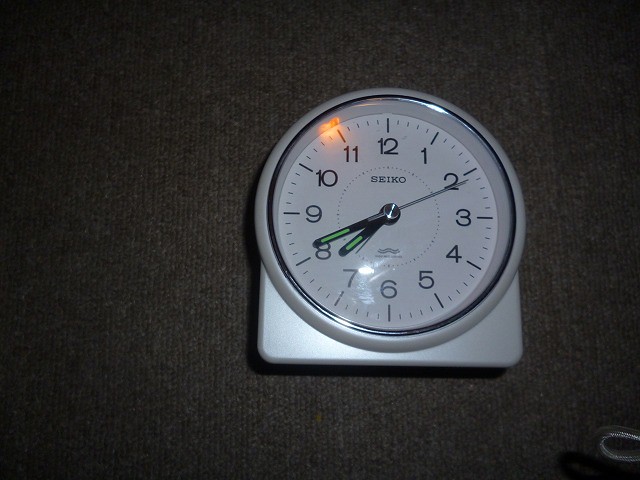The image features a prominently displayed white analog Seiko clock set against a dark, textured fabric, possibly a carpet that appears gray but could have dark taupe tones. The clock is positioned slightly to the right-center of the image, with its frame designed to include a square stand at the bottom. This design choice allows the clock to either stand upright or add a unique touch to its appearance. The clock face itself is primarily white with black numbers 1 through 12, supplemented by dashes representing seconds and additional circular black dot markings. The slim black minute and hour hands are accented with green, while the second sweep hand is silver. The brand name, SEIKO, is prominently displayed beneath the number 12. A gray cord with a hoop shape is partially visible in the bottom right-hand corner of the image, adding to the overall detail of the scene. The time shown on the clock reads approximately 7:41.